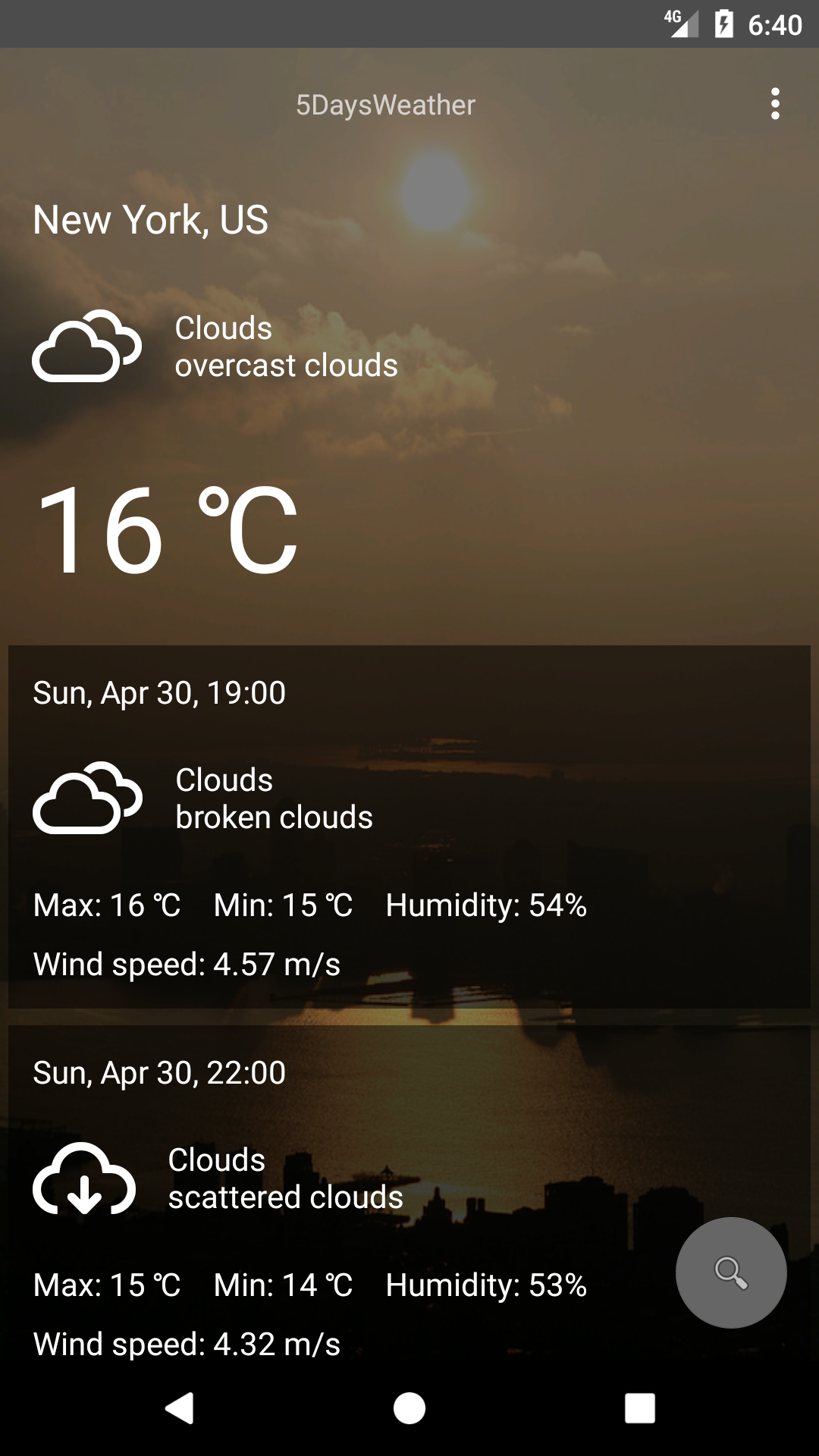A screenshot of a smartphone's weather app interface is displayed. The top edge of the screen features a black background with various status icons: battery charging, signal bars, and the time, 6:40. Below this, a five-day weather forecast is shown against a dark, ocean-like background that is partly obscured and difficult to discern clearly.

The weather information detailed for New York, US, features overcast clouds with a current temperature of 16 degrees Celsius. More specific data includes the date, Sunday, April 30th, and time, 19:00, alongside descriptors like "clouds broke in clouds," a maximum temperature of 16 degrees Celsius, a minimum of 15 degrees Celsius, 54% humidity, and a wind speed of 4.5 m/s. 

For Sunday, April 30th at 12:00, the forecast mentions scattered clouds, a maximum temperature of 15 degrees Celsius, a minimum temperature of 14 degrees Celsius, 53% humidity, and a wind speed of 4.32 m/s. 

The bottom portion of the screen shows navigation icons: a back arrow, a circle, and a square, all set in white font. A gray circle with a magnifying glass icon is located in the lower right corner. The overall color scheme of the interface includes brown and black tones, and there appears to be an overlay filter on the background, making the underlying photo difficult to see clearly.